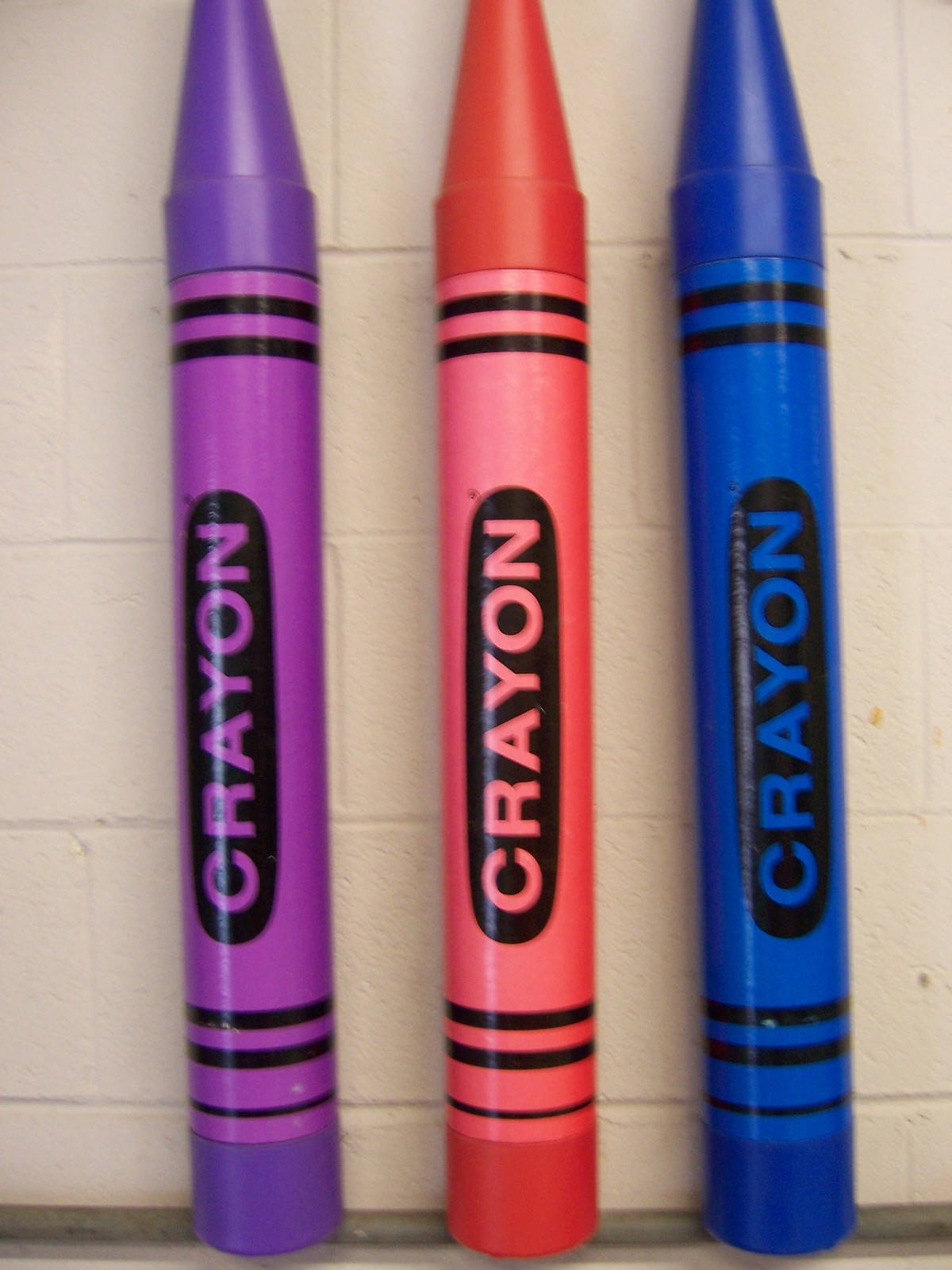This is a digital photograph taken indoors featuring three oversized, comically large crayons that resemble piggy banks, though that part is not fully visible. The crayons are positioned vertically against a cinder block wall painted white. The floor and the gray running strip at the base of the wall are of the same color, seamlessly blending together. The crayons are colored purple, orange, and blue from left to right. Each crayon bears the word "crayon" in black letters within a black oval outline, corresponding to their respective colors. At both the top and bottom of each crayon, there are two thick black horizontal stripes and a thinner one near the end, mimicking the typical design of crayon wrappers.